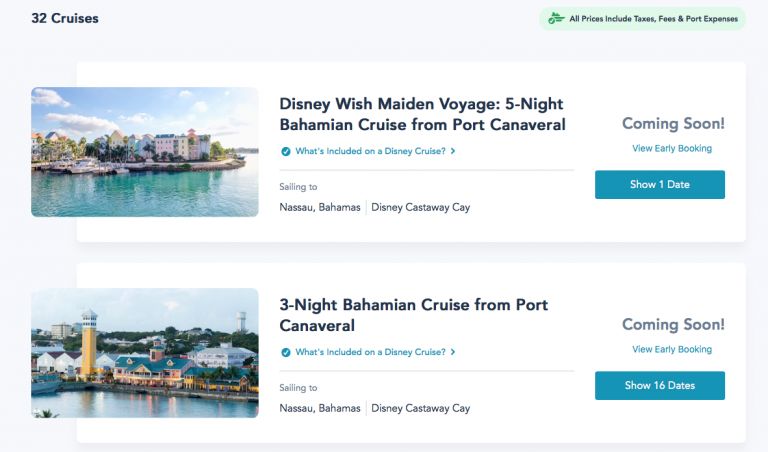This website specializes in cruise vacations and highlights 32 available cruises, prominently displayed in black text against a gray background. To the right, there's a light green button indicating that all prices include taxes, fees, and port expenses.

Visible on the page are two featured cruises. The first is the **Disney Wish Maiden Voyage: Five Nights Bahama Cruise** departing from Port Canaveral. Clicking on the details reveals that the cruise will visit Nassau, Bahamas, and Disney's Castaway Cay. It also mentions early booking opportunities and has an image associated with Castaway Cay, showcasing a serene landscape with clear blue skies, turquoise waters, and vibrant buildings. The predominant colors in the image include shades of black, teal, green, gray, white, yellow, blue, and brown.

Beneath this, there is the **Three Nights Bahama Cruise** also departing from Port Canaveral. Details for this cruise include stops at Nassau, Bahamas, and Disney's Castaway Cay, similar early booking options, and 16 available departure dates. This section also features an image of Disney Castaway Cay, which likely emphasizes the picturesque scenery of water, sky, and shoreline. The colors seen here are consistent with the overall theme: black, teal, green, gray, white, yellow, blue, and brown.